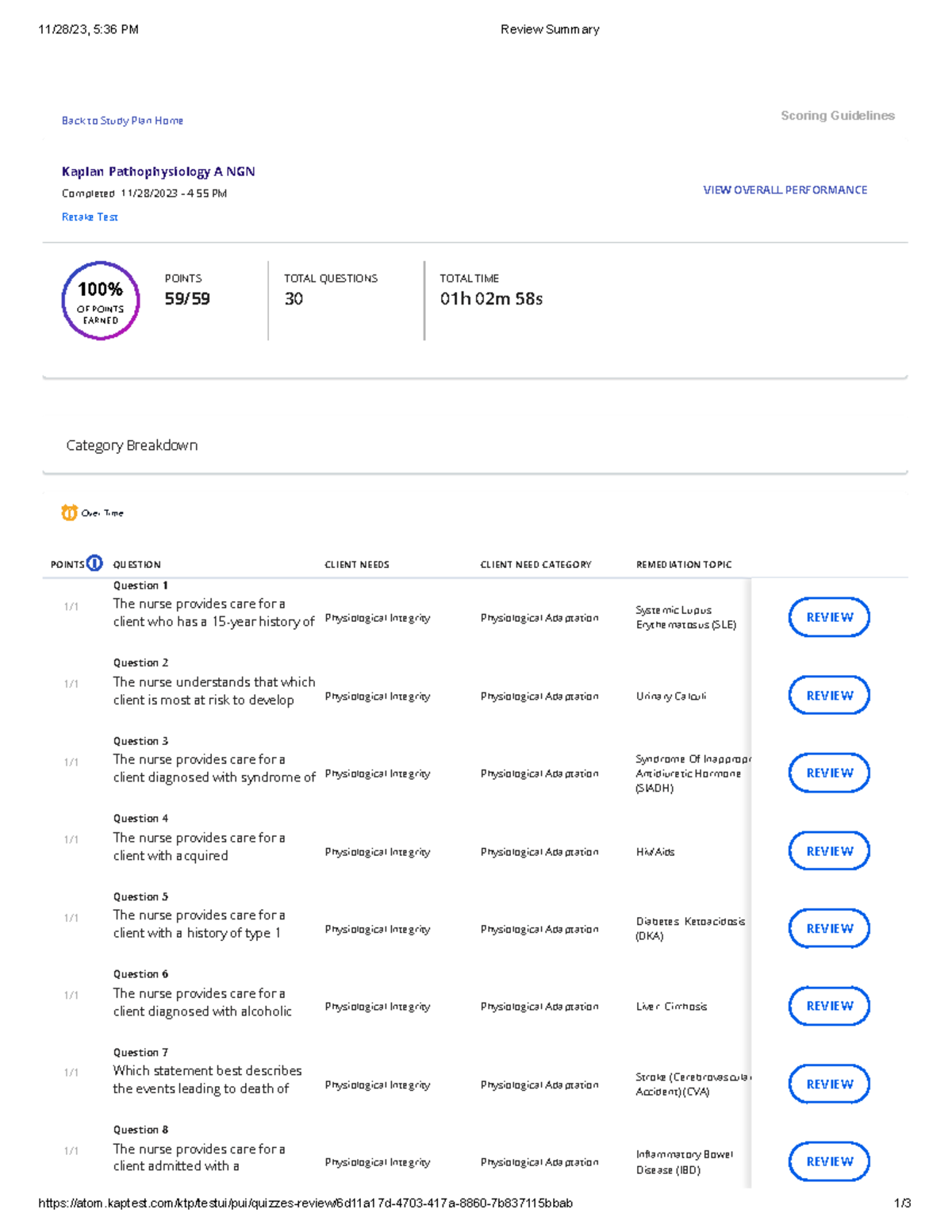This screenshot captures the results page of a Kaplan Pathophysiology practice test, specifically tailored for the medical and nursing fields. The image is vertically oriented, making it taller than it is wide.

In the upper right-hand corner, there is a "Scoring Guidelines" label, while the upper left-hand corner features a "Back to Study Plan Home" button. Below that, it reads "Kaplan Pathophysiology A NGN completed 11/28/23 at 4:55 PM." There is also an option to retake the test.

The examinee achieved a perfect score: 59 out of 59, with 100% points earned from a total of 30 questions. The duration of the test was 1 hour, 2 minutes, and 58 seconds.

The "Category Breakdown" follows, listing the questions along with the points earned. For each question, the person scored one out of one, indicating a perfect response rate. The beginning of each question is provided for context, for example, "Question 1: The nurse provides care for a client who has a 15-year history of...".

The columns are labeled as follows:
- "Client Needs"
- "Client Need Category" (which is consistently "Physiological Adaptation" for all questions)
- "Remediation Logic"

The first row specifically mentions "Systemic Lupus Erythematosus (SLE)" under the "Remediation Logic" column.

Additionally, there is a blue button available on the screen to review any questions that might have been answered incorrectly, although in this case, no such review is needed since the examinee scored perfectly.